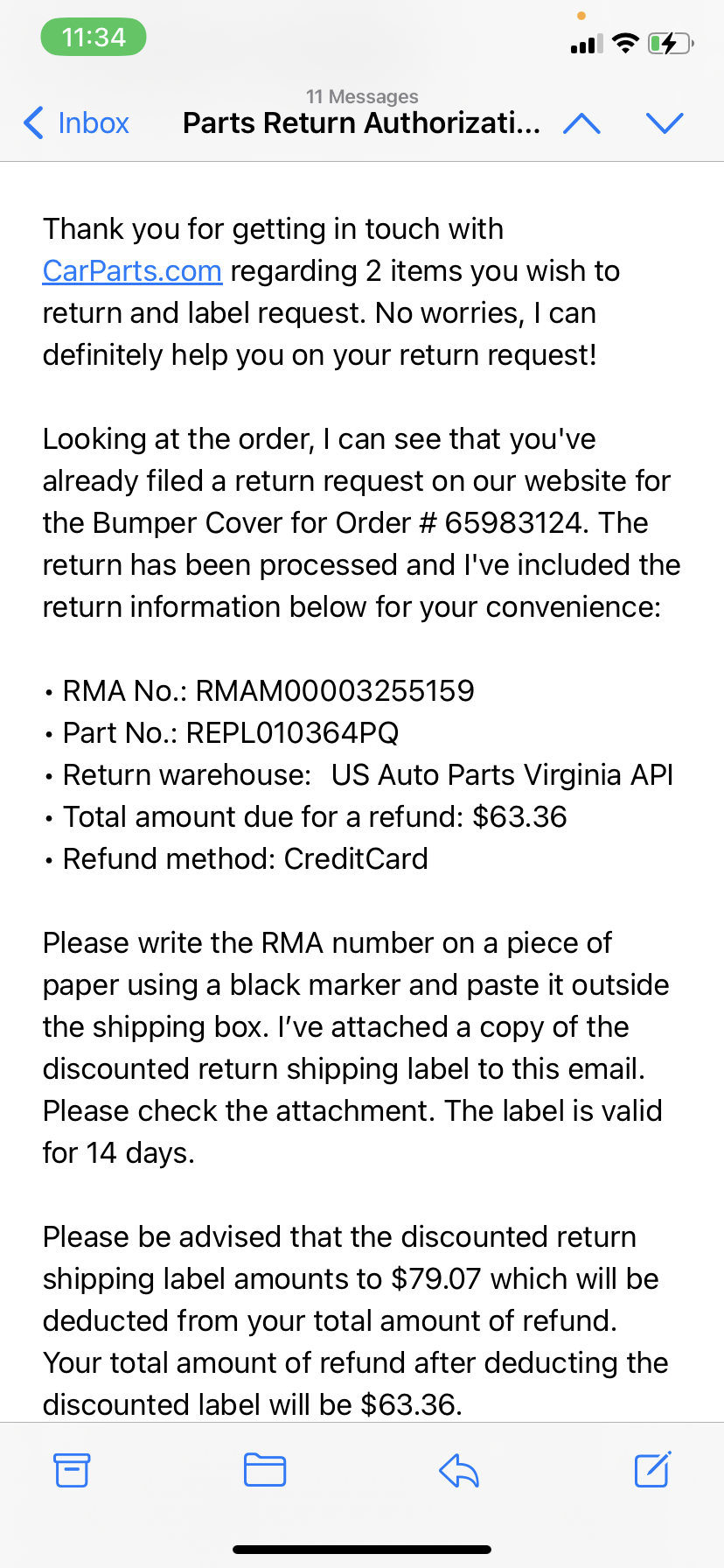A detailed information page is displayed, resembling a messaging app interface. The top left corner features a green time bubble displaying "11:34." In the top right corner, indicators show "3 of 4" for data, "3 of 3" for Wi-Fi, and a battery charging icon. The main content area is titled "Inbox: Parts Return Authorization" with an additional note of "11 messages" indicated by blue up and down arrows.

The message content begins with a greeting and thanks the recipient for contacting CarParts.com regarding the return and label request for two items. The representative assures assistance with the return request, mentioning that a return request for a bumper cover, associated with order number 65983124, has already been processed on their website. 

Detailed return information is provided: 
- RMA Number: RMAM00003255159
- Part Number: REPL010364PQ
- Return Warehouse: US Air Auto Parts Virginia API
- Total Refund Amount: $63.36
- Refund Method: Credit Card

Instructions are given to write the RMA number on a piece of paper using a black marker and affix it to the outside of the shipping box. An attachment is included in the email containing a discounted return shipping label. The label is valid for 14 days, and it is noted that the cost of the return shipping label—$7.90—will be deducted from the total refund amount, leaving a net refund of $63.36.